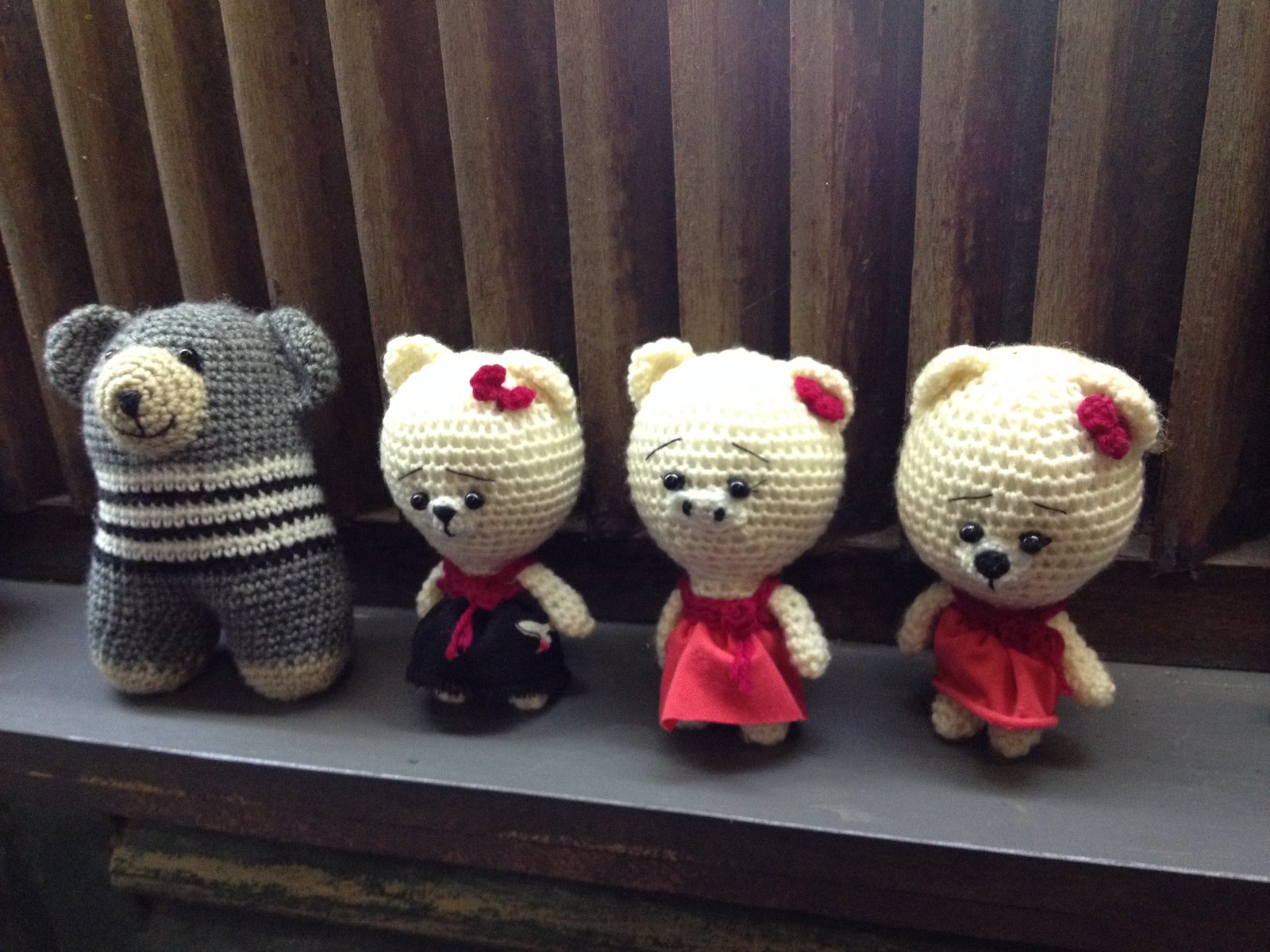The color photograph features a worn, scratched, and faded gray wooden cabinet. On top of the cabinet are four hand-crocheted animals, each displaying unique characteristics and charming details. The first character is a gray bear adorned with a tan nose and paws, and it sports white and blue stripes around its neck, resembling a scarf. Next, there is a set of three animals crocheted from white or off-white yarn: the middle one appears to be a pig, while the others are bears. All three are dressed in little outfits and have oversized, rounded heads, akin to bobbleheads, with crocheted red flowers in their left ears. The attire of these three includes red dresses with bows, enhancing their endearing, handcrafted appeal. The meticulously made crochets possess a whimsical allure, suggesting they might be displayed either for sale or as part of a personal collection.